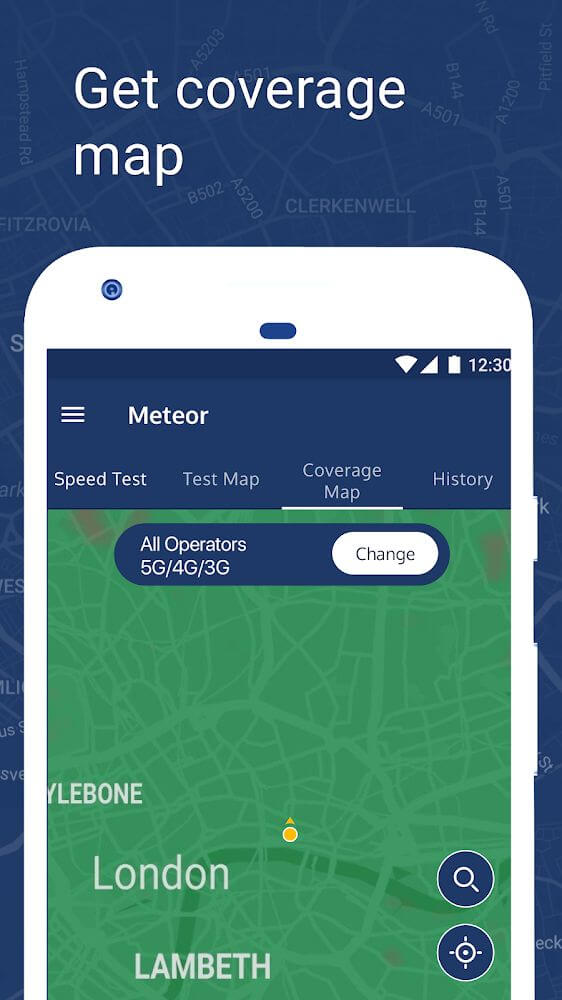A detailed screenshot of a phone screen displays a map interface. The background features another dark blue map. At the top of the screen, white text reads "Get Coverage Map". The phone graphic itself is white with a blue top bar labeled "Meteor". Below the top bar, there are four links: "Speed Test," "Test Map," "Coverage Map," and "History." Next, there's a dark blue, pill-shaped section labeled "All Operators 5G/4G/3G" with a white pill-shaped button beside it saying "Change". The main map displayed in green covers the London area, indicated by the label "London" in the bottom left corner. In the bottom right corner of the screen, there are three dark blue circle icons: a magnifying glass, a crosshair, and a rectangle.